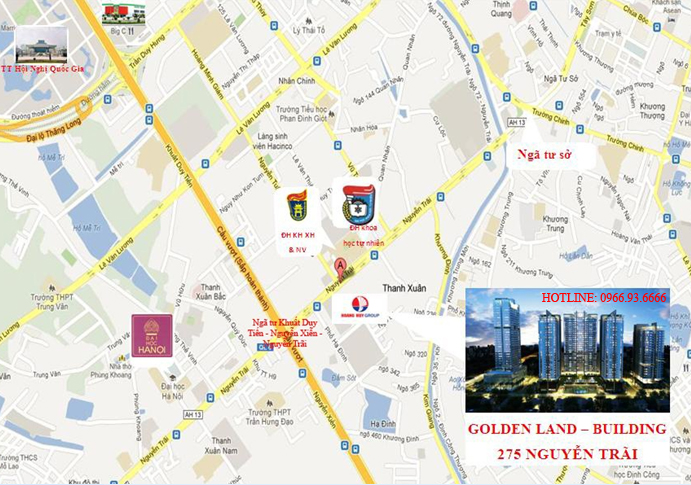This image is a detailed close-up view of a map, likely from an online map application, depicting either a region in China or Vietnam. The map features various roadways indicated by orange and yellow lines on a gray background. Different areas are color-coded, showing green spaces, blue water bodies, beige zones, and white streets. Street names are written in black letters for clarity. Notable locations are marked with white icons that include a logo and explanatory text in Vietnamese. In the bottom right-hand corner, there is an inset image of skyscrapers with the text "Hotline 0966 93 6666" in red. Below this image, the caption reads "Golden Land Building, 275 Nguyen Tri."